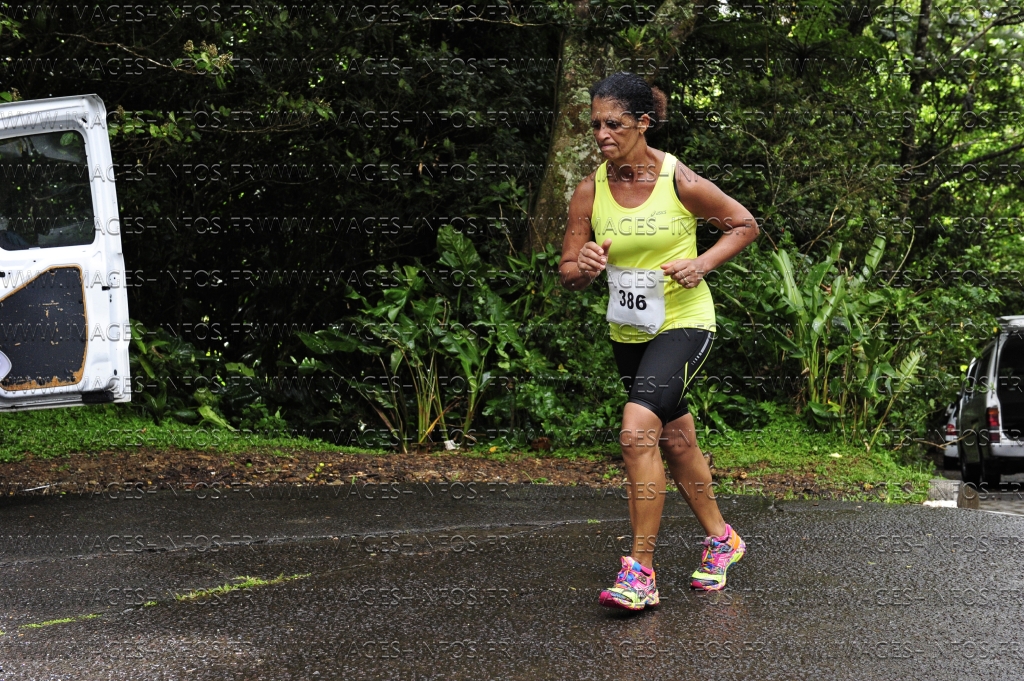In the foreground of this landscape photograph, a middle-aged woman with a darker complexion, possibly of Indian descent, is seen jogging towards the camera at a 45-degree angle from right to left. She has slicked-back black hair, styled in a bun, and is dressed in a lime green tank top with the number 386 displayed on a white paper pinned to her chest. She pairs this with black spandex biker shorts and vibrant pink and blue running shoes. The woman's expression is one of determination, her face set in a grimace. She is running on damp pavement, which appears wet, suggesting recent rain. The background is lush with forest greenery, including trees, bushes, and tropical plants. Alongside the road, there are parked cars with their trunks open, one visible on either side of the image.